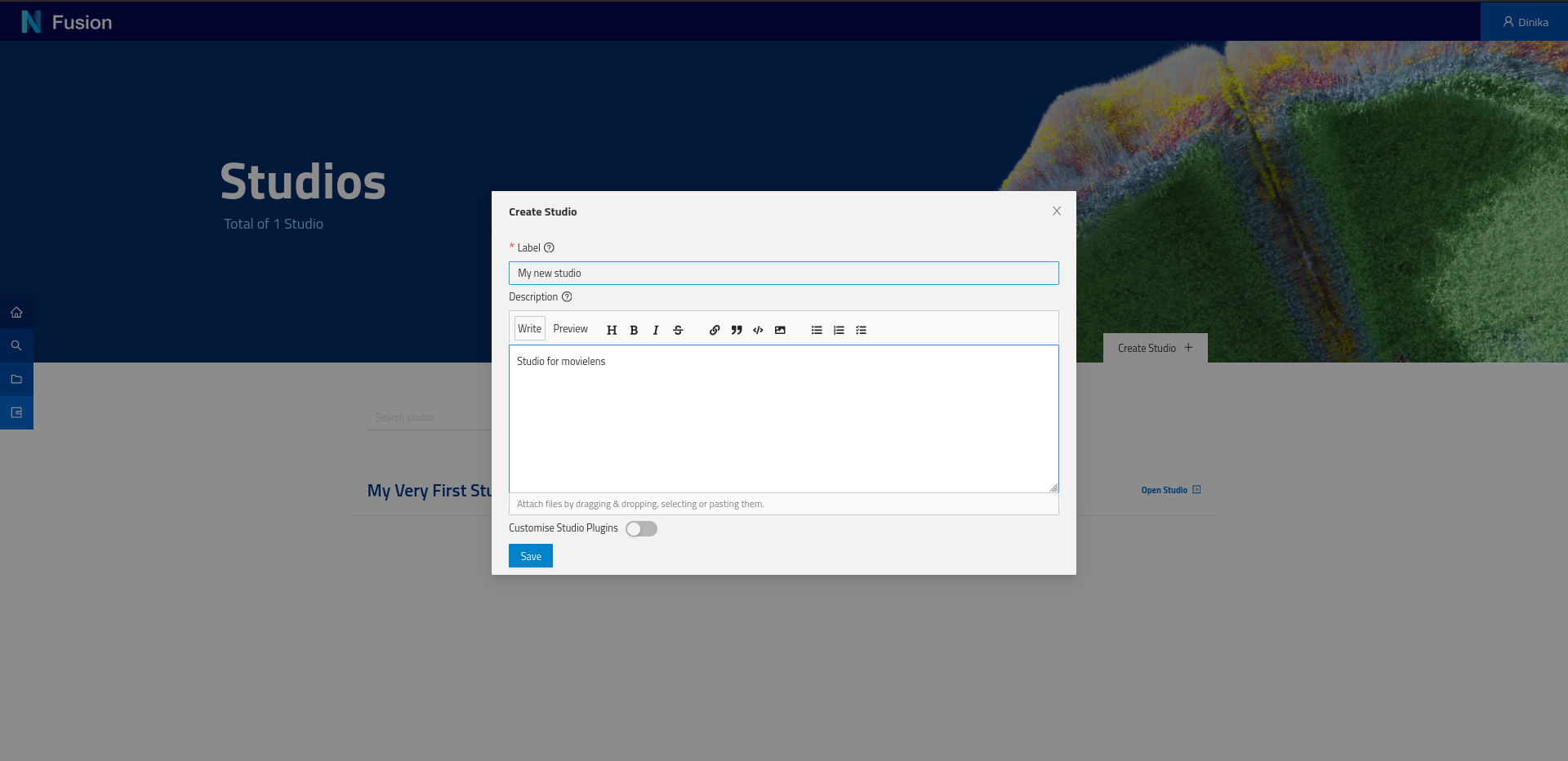On a web page with a dark-themed design, a light gray pop-up window is prominently displayed. The pop-up’s header features gold and black text reading "Create Studio." Below that, a gray section with a red star icon contains the word "Label" alongside a circular question mark icon. A blue-bordered rectangle within this section displays the phrase "My New Studio." Underneath it, a "Description" label, also accompanied by a question mark icon, precedes a white text rectangle with the words "Studio for movie lens."

Above this, a set of tabs is present, with the "Write" tab selected. Additional tabs include "Preview," "Bold" (denoted by 'B'), "Italic" (represented by a tilted 'I'), "Strikethrough" (indicated by an 'S' with a line through it), and other formatting icons such as link insertion, quotation insertion, and code snippets (shown as '< / >'). Options for text alignment (left, center, right) and bullet points with checkmarks are also visible.

Outside the content area, a light gray rectangle invites users to "Attach files by dragging and dropping, selecting, or pasting them." This rectangle stands out against a darker gray background, which features a deactivated "Customized Studio Plugins" slider. The slider consists of a white circle on a dark gray track, indicating its deactivated state.

On the lower left corner of the pop-up, a dark blue rectangle with the word "Save" in white is available for saving changes. 

In the background, the top of the page has a dark purple or dark blue bezel containing the word "Fusion" in a gradient of cyan blue to white, followed by the bold white text "Studios." Beneath it, cyan blue text states "Total of one studio." 

A bezel along the left side of the page transitions from dark blue to lighter blue and displays icons for Home, Search (magnifying glass), Folders, and what appears to be a Presentation. 

On the right side of the screen, a multicolored design resembling a sea creature is visible. This design transitions from yellow and beige at the top to a mix of pink and blue, eventually becoming predominantly green with blue and pink bands.